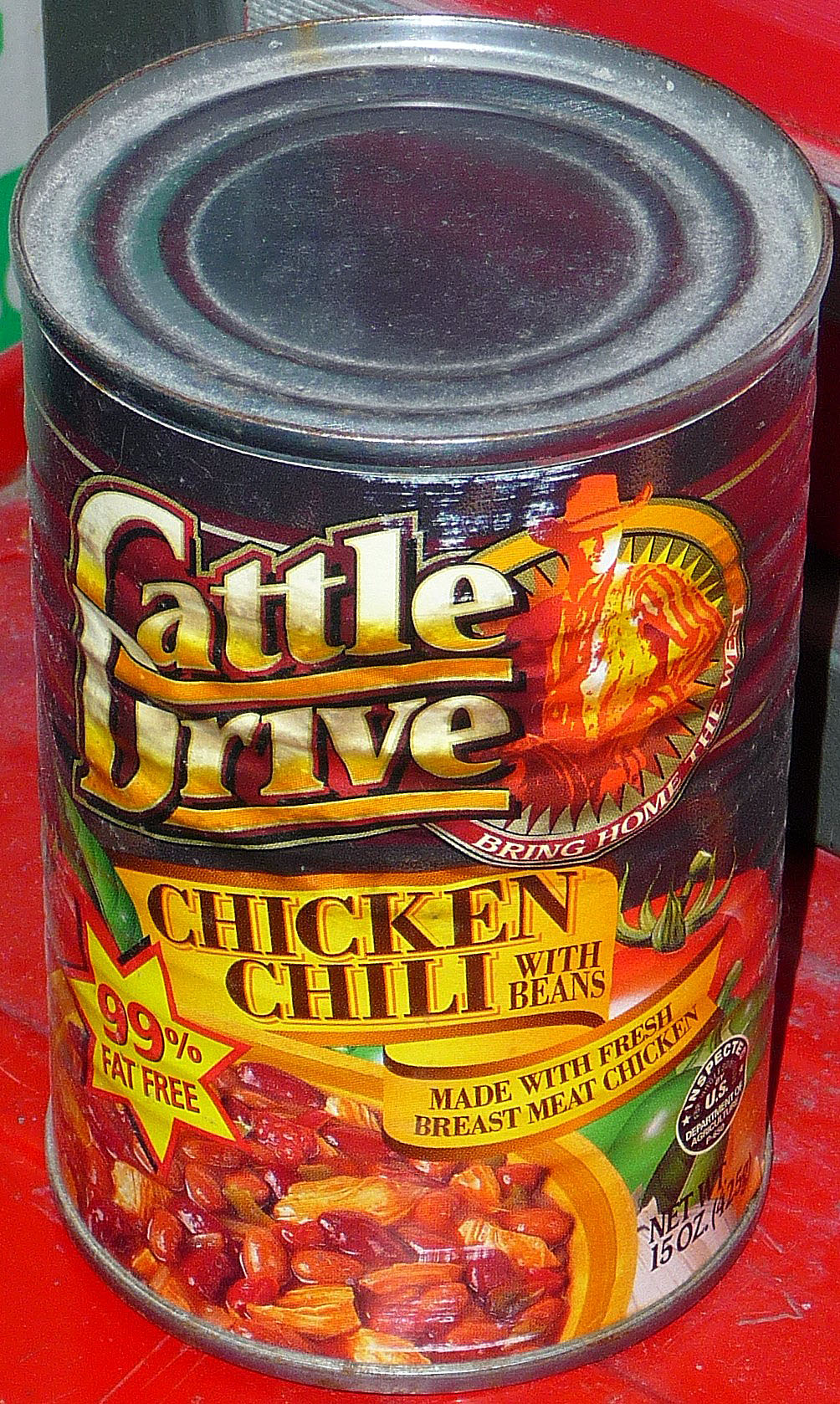This close-up photograph features a can of "Cattle Drive Chicken Chili with Beans," prominently labeled as 99% fat-free and made with fresh breast meat chicken. The can displays a U.S. inspection mark, and at the bottom in black ink, it specifies a net weight of 15 ounces (425 grams). The bottom left corner showcases an appetizing picture of the chili in a yellow bowl, revealing beans, peppers, chunks of chicken, and onions.

At the top of the can, the "Cattle Drive" brand logo is visible, accompanied by a circular logo depicting a cowboy with his hands on his hips, looking to the right, encased in a medallion-style design. Below this logo, white lettering reads, "Bring Home the West."

The can itself appears somewhat aged and dusty, with noticeable dust buildup around the ridges at the top. It is positioned on a red, dusty surface, enhancing the vintage and rustic feel of the image.